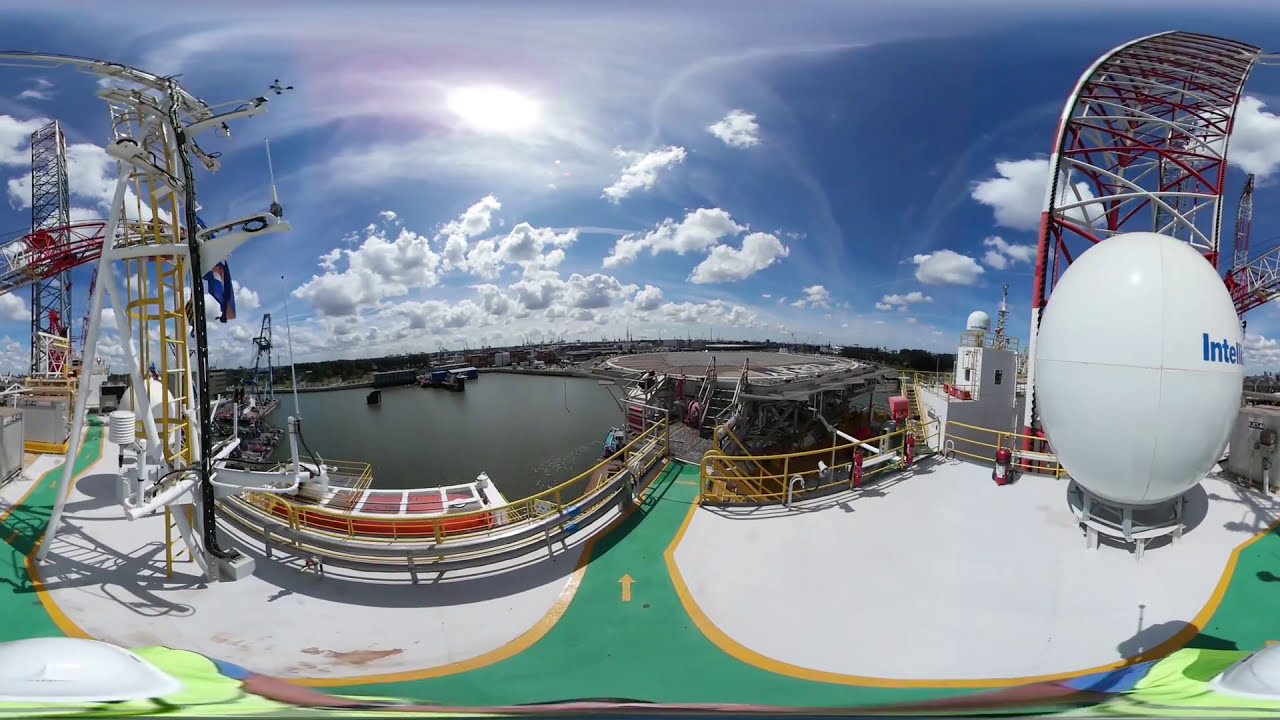The photograph, taken outside on a clear day, captures a panoramic view of a bustling harbor area beneath a beautiful blue sky scattered with fluffy white clouds. The sun peeks through the clouds toward the upper middle of the photo, illuminating the scene with a gentle glare. Prominently featured is a sprawling ship or barge equipped with a crane system, characterized by its white walkways bordered in yellow and bisected by green pathways. Metal structures and towers, painted red and white, rise above the ship, with one larger tower to the right and another tall one to the far left.

Central to the photo is a walkway leading out to a round concrete platform, reminiscent of a helicopter pad, accessible by stairs. A notable feature on the walkway is a large, white, egg-shaped object, likely a satellite dome marked with the partially visible word “INTELL.” Two white circles with yellow outlines are also visible on the deck.

In the background, the harbor is defined by a murky body of water, beyond which lies a distant cityscape interspersed with trees and buildings, adding to the industrial yet picturesque setting. The scene is bathed in bright daylight, emphasizing the intricate details and the vibrant colors present throughout the image.